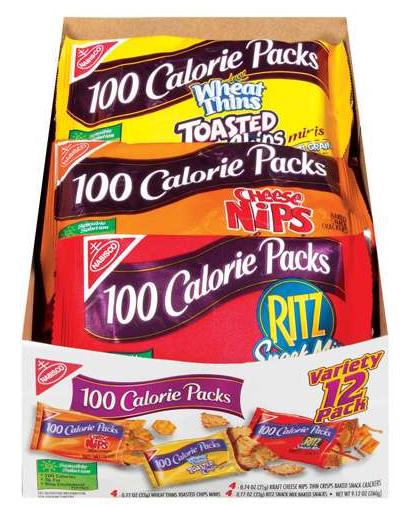This product photograph showcases a variety pack box containing different types of crackers, specifically 100-calorie packs from well-known brands. Arranged in the image, the rear package features Wheat Thins in a yellow-colored wrapping. Positioned in front of the Wheat Thins is an orange 100-calorie pack of Cheese Nips. At the forefront, there is a red bag of Ritz crackers. The front of the box prominently advertises that it is a 12-pack variety set, offering an assortment of the previously mentioned brands in convenient, single-serving 100-calorie packages.